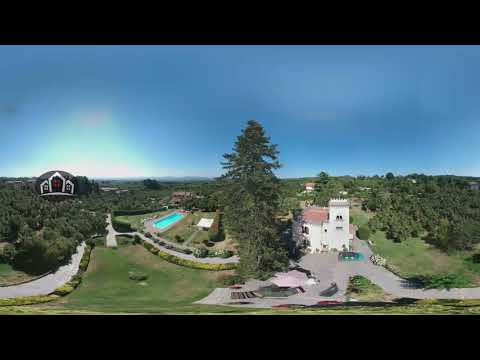In this high-angle, panoramic shot, likely taken by a drone, a large, dark green evergreen tree stands prominently in the center of the image. To the right of this towering tree is a white brick building with a striking red roof. This building features two upper and two smaller lower windows, with one section on the right rising slightly taller. A long gray driveway leads to this house, curving behind the tree and extending towards another building in the background. This distant structure, with its arch shape and red walls outlined in white, sits against a backdrop of light colors that merge into a blue sky.

To the left of the central tree lies a swimming pool, its water a light teal color. The pool is flanked by a patchy field of grass, a mix of browns and greens, and surrounded by shrubs in varying shades of green. Nearby, a large grassy courtyard area can be seen. In the background, beyond the house and the courtyard, a few trees and additional buildings are visible. The image has a slight distortion due to the panoramic view, and some details appear grainy, suggesting a lower resolution.